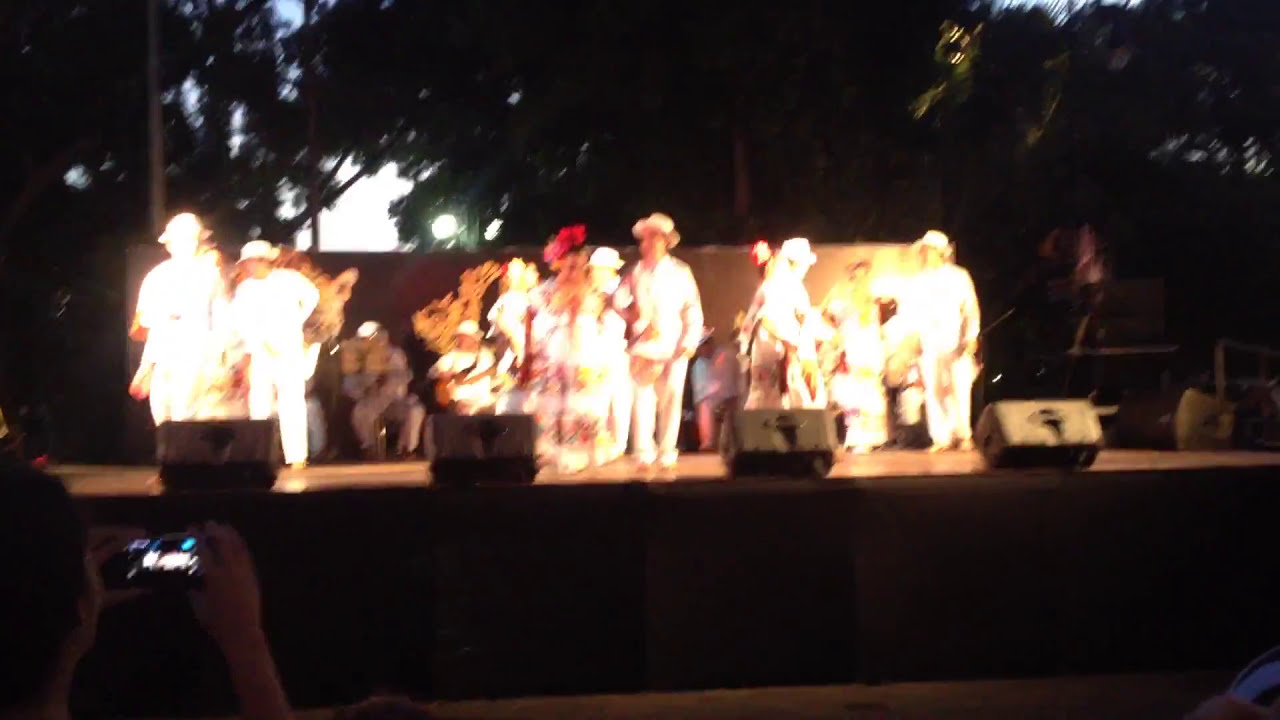The photograph captures an outdoor stage performance set around dusk, featuring at least 12 performers who appear as blurry, glowing orbs of light due to the flash. The raised stage has four speakers mounted at the front, and despite the distortion, some performers seem to be wearing white outfits, with men in hats and women possibly adorned with flowers. The scene is framed by tall trees that stand silhouetted against the darkening, blue-hued sky. In the bottom right corner of the image, an audience member can be seen holding up a device to record the event. The twilight setting creates a balance between the fading daylight and the artificial lighting focused on the stage, enhancing the overall atmosphere of a lively park performance.